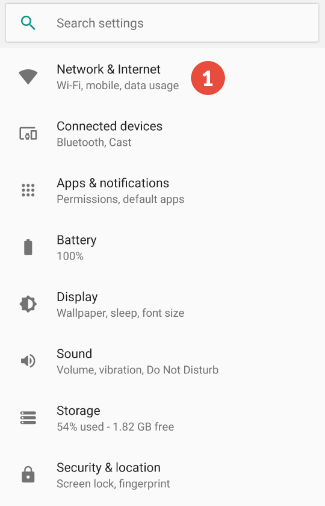Screenshot depicting the settings menu of an Android phone. At the top, there is a standard search bar labeled "Search settings." Below, various categories are listed: "Network & Internet" including sections like Wi-Fi, Mobile, and Data Usage; "Connected Devices" covering Bluetooth and Cast; "Apps & Notifications" featuring Permissions and Default Apps; "Battery" displaying a full 100%; "Display" with options for Wallpaper, Sleep, and Font Size; "Sound" containing adjustments for Volume, Vibration, and Do Not Disturb; "Storage" indicating 54% usage with 1.8 GB free; and "Security & Location" highlighting options for Screen Lock and Fingerprint. Notably, a red circle with a white number '1' is present to the right of the "Network & Internet" category, suggesting a notification or alert.